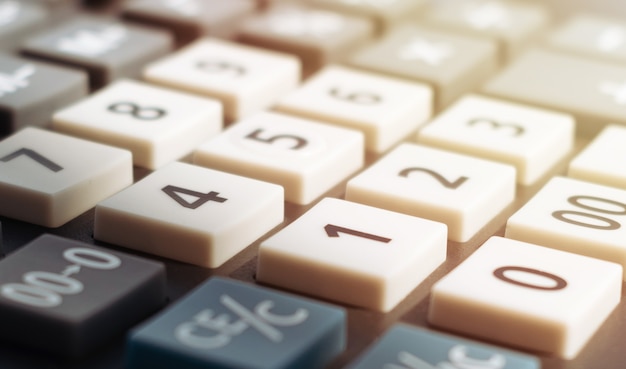This photograph features a close-up of an old calculator or peripheral keyboard keypad, prominently showcasing a grid of raised, cream-colored keys with brown numerical and symbolic inscriptions. Centered within the image, the keys are arranged in a familiar numeric keypad layout often found on the right side of keyboards. The numbers ascend from bottom to top: 0, 00 at the lower right, followed by rows of 1-3, 4-6, and 7-9.

The keys exhibit minor shading variations, appearing darker on the left side. Notable keys include two blue keys labeled "CE/C" and an unclear label beneath it, which is partially visible due to being a bit out of focus. Another black key on the middle left bears the label "00→0" in white font. Additional, partially visible keys above these are in muted colors like gray, dark green, and brown, hinting at functions for fractions or percentages, typical of calculators from the 1990s or early 2000s. The keys' distinct color contrast and old-fashioned design evoke a sense of nostalgic practicality, reminiscent of an era before sleek modern interfaces.